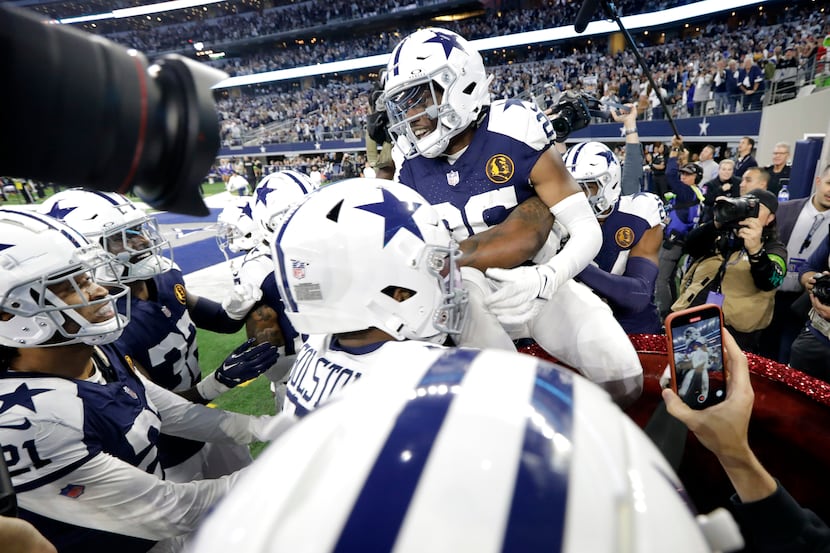In this image of a jubilant scene at the Dallas Cowboys Stadium, the focus is on a spirited celebration following a victorious football game. The stadium is packed with cheering fans, indicated by the stars decorating the background stands. Players in navy blue jerseys with white numbers and shoulders marked by blue stars are gathered closely, showcasing their white helmets accented with navy blue stars and stripes. One player, held aloft by a teammate gripping his waist, stands out smiling, suggesting he may have scored the game-winning play. A sea of arms holds up mobile phones recording the celebratory moment, with a noticeable iPhone displaying a red recording button. To the left, a large professional camera captures the scene, and above, a long pole-mounted microphone hangs, ready to catch the joyous noise of the crowd. This detailed snapshot captures the essence of a victorious and exuberant post-game celebration.